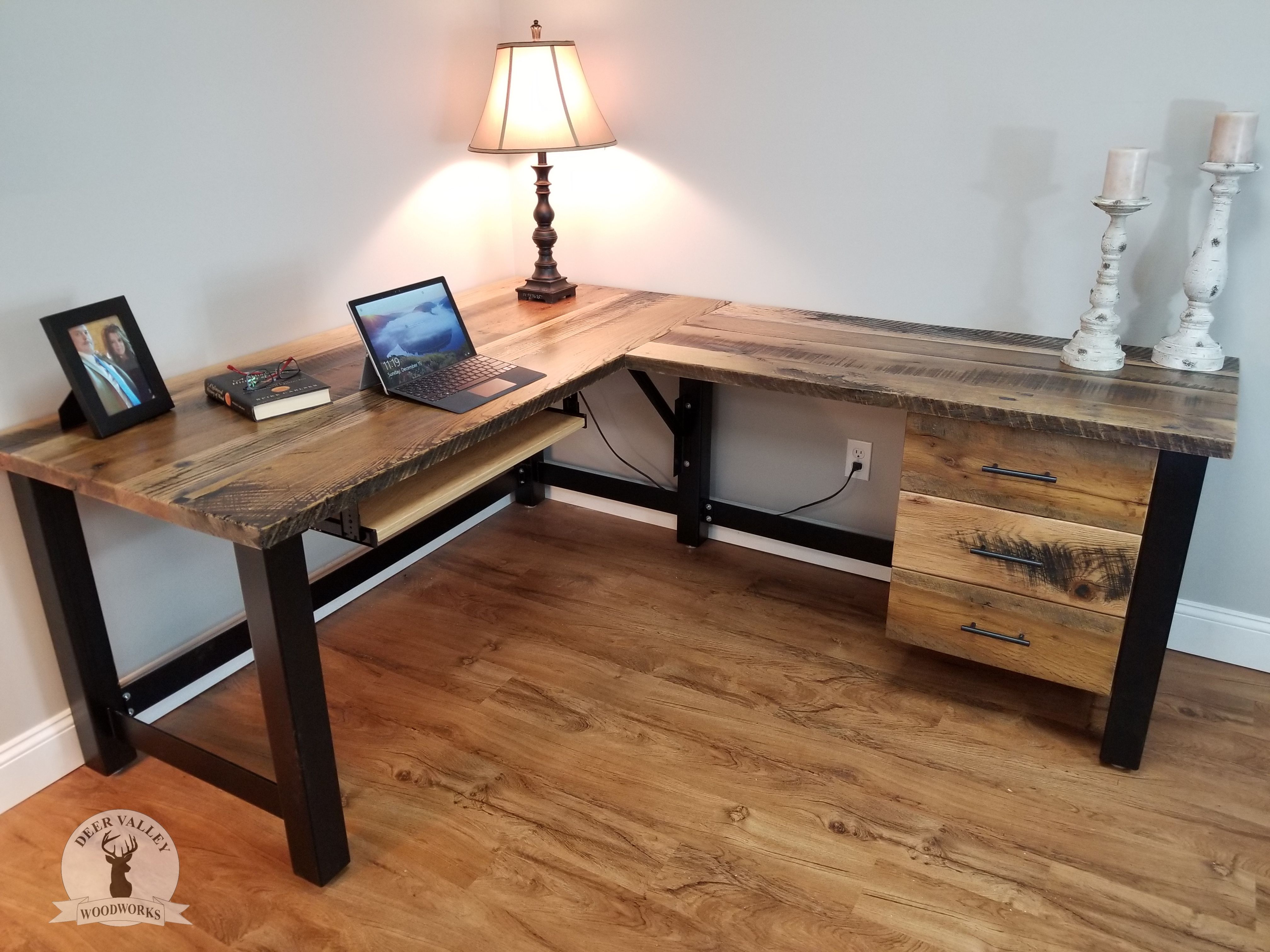This professional photograph showcases an L-shaped wooden desk perfectly nestled into the corner of a room. The desk features a harmonious combination of a light brown wooden top and drawers, complemented by sleek black metal legs and beams. The flooring beneath is a light brown wood pattern, adding to the warm ambiance, and is bordered by a white baseboard above it. 

On the desk, a small laptop is positioned centrally, flanked by personal touches that enhance the workspace's aesthetic. On the left side, a neat picture frame displays an image of two individuals, possibly siblings or friends, with the backdrop of the 80s style. A book sits beside this, topped with red-framed glasses, ready for a quick read. In the corner stands a classic lampshade with a dark brown base, casting a soft, pleasant light over the area. To the right, two elegant decorative candles add a touch of sophistication.

Below the desk's surface, three wooden drawers offer storage solutions, designed in a similar light brown wood finish to maintain a consistent look. Next to the drawers, a pull-out shelf is available, probably intended for a keyboard. The background wall is a soothing light gray, adding a subtle contrast that highlights the desk's details.

Adding a finishing touch to the image, the bottom left corner proudly displays the logo of Deer Valley Woodworks, featuring deer antlers and the company's name in a white circular backdrop, emphasizing the craftsmanship and brand identity involved in creating this beautiful workspace.